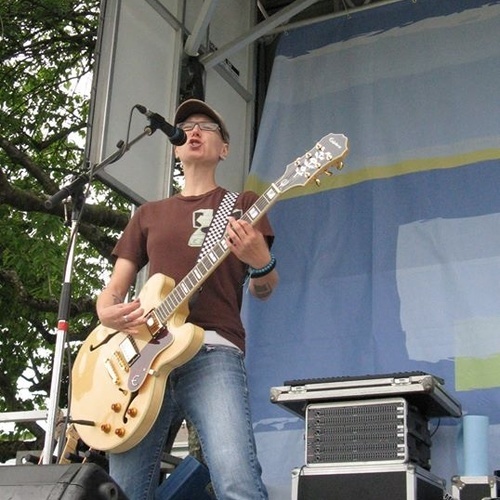The image captures an outdoor concert scene with a single white man on stage, playing a yellow electric guitar and singing into a black microphone. He is dressed in a brown short-sleeve shirt featuring a yellow graphic, faded blue jeans, and a brown cap. He is also wearing brown glasses, a black bracelet, and a gold ring on his right hand, which holds a guitar pick. His left hand, adorned with a gray and black tattoo, is positioned on the top strut of the guitar. The man stands under an awning with a sound amplifier behind him. The background reveals a stage backdrop in pale blue and yellow colors, along with lush greenery including a large tree with many branches and green leaves, suggesting a park-like setting. The overall ambiance hints at a possibly cloudy day, making it a typical "music in the park" event.